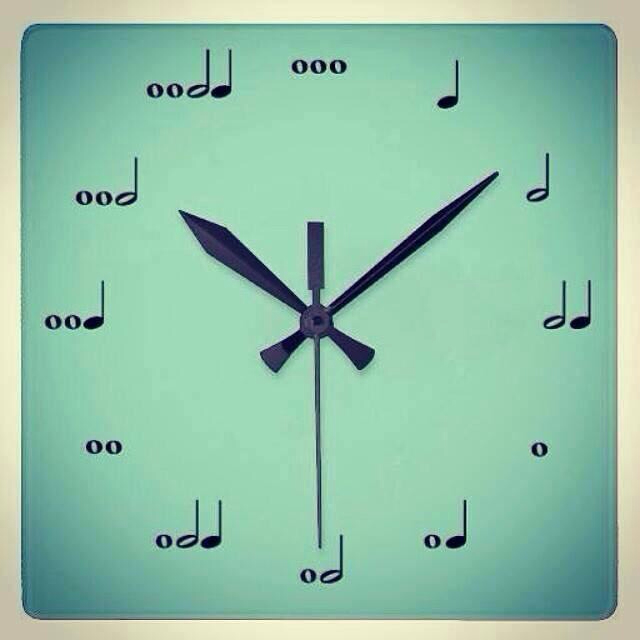The image features an indoor, square-shaped analog clock with a unique twist: instead of traditional numerals, musical notes are used to represent the hours. The clock face is a light green color, transitioning to a slightly darker shade towards the corners, giving it a subtle gradient effect. The outer border is a light cream color, blending seamlessly into the clock's design or possibly resting on a white surface.

At the 12 o'clock position, there are three circles with white spots in the center, marking it uniquely. At 1 o'clock, there's a crotchet (a solid oval note), and at 2 o'clock, there's a minim (a note with an open circle). The 3 o'clock position features two musical notes (one solid and one with a white center), while at 4 o'clock, there is just a circle with a white spot. This pattern continues around the clock, with each hour represented by various musical notation and note combinations.

The clock's hands are black; the hour hand points towards the 10 o'clock position, the minute hand between the 1 and 2 o'clock positions, and the second hand at the 6 o'clock position, indicating a time of about 7 minutes past 9. This clock is not only functional but also a creative and artistic piece, with no additional text or markings on its face, making it a unique and visually appealing timepiece.